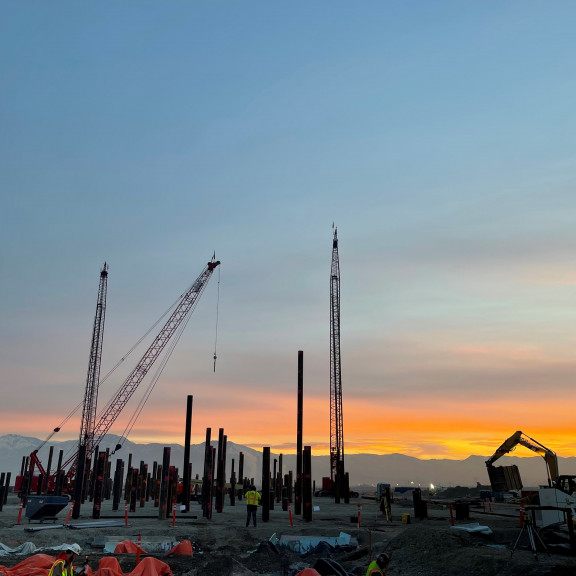This color photograph, taken at either sunrise or sunset, captures an active construction site bathed in an orange glow from the horizon. The sky transitions from blue to purple with scattered orange clouds. Dominating the scene are three towering cranes and numerous tall, dark columns made of rebar or metal, designed to support a future building or skyscraper. The site is filled with industrial tools, machinery, and bright orange tarps. In the foreground, one worker is digging in a large dirt pile, while another stands in the center with his back to the camera, distinguishable by his high-visibility yellow and orange safety vest. The ground is mostly dirt, and the overall atmosphere suggests early morning activity.